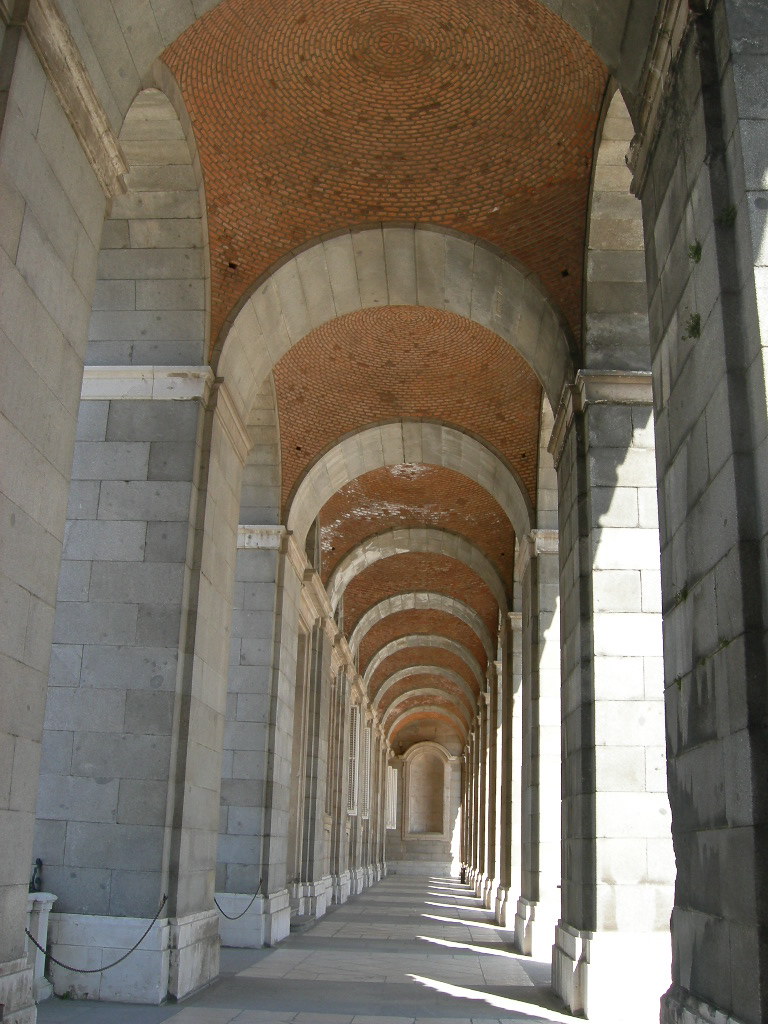The photograph depicts a long hallway formed by a series of approximately six to seven cement block archways, which create an illusion of a tunnel. The archways extend from the foreground to the distant background, converging towards the center of the image. The cement block pillars, which are light to dark gray in color, support the structure on both sides. Above, the ceiling is composed of red bricks arranged in an arch formation, adding a historic texture to the scene. Sunlight streams in from the right, illuminating sections of the pillars and a portion of the ground, which is also cement and varying in shades of gray. At the far end of the hallway, there is an enclosure that could be a window or a niche, often found in religious or historical buildings. The image evokes the atmosphere of an ancient site or a popular tourist location, emphasizing the timeless beauty of the architectural design.